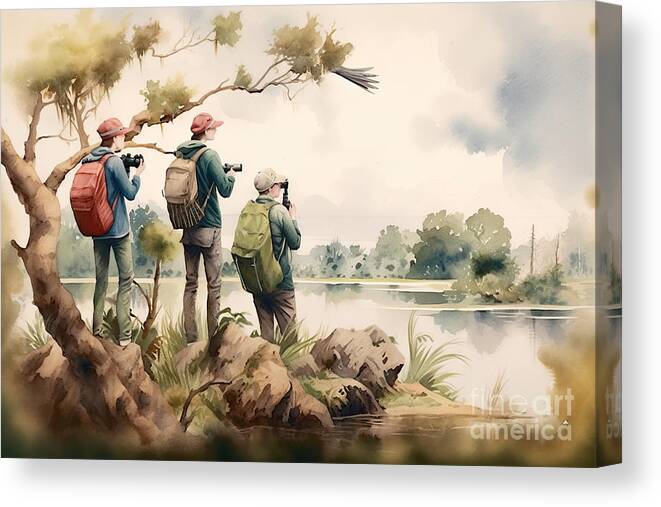The image is a detailed watercolour painting on a rectangular, block canvas with no frame, rendering a vivid scene at the shore. In the foreground, three young, slender men stand with cameras in hand and backpacks on their backs, each wearing caps. They are positioned on the left side of the painting with their backs to the viewer, gazing intently across a serene lake towards the right. The leftmost man has a red backpack, a blue shirt, and grey pants; the middle man sports a grey backpack, a green jacket, and nearly black pants; the rightmost man carries an olive green backpack and wears a somewhat blue jacket with slightly black pants. A tree with a brown trunk and green leaves stands behind them to the left, while rocks scatter the ground beneath their feet. The scene is framed by a mostly white sky with hints of grey, and the middle ground features a tree line extending across the entire width of the lake. The lake itself lays placidly between the sky and the shore. Additionally, there is faint watermark text on the bottom right, reading "Fine Art America," indicating the artwork's origin. The solid white background of the canvas enhances the vivid colors of the landscape and the figures within, offering a striking, immersive viewing experience.